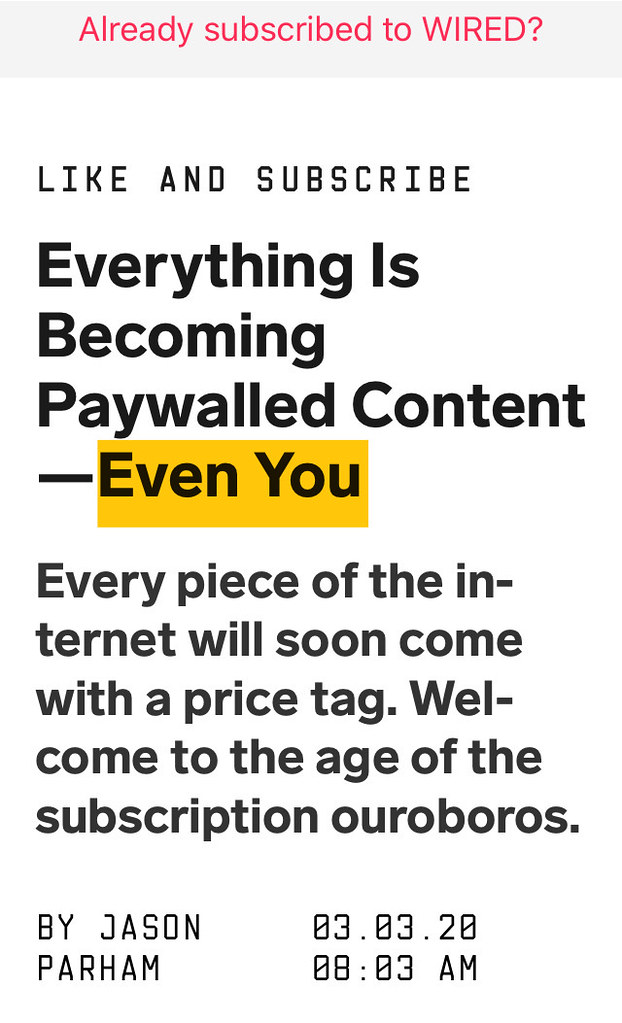The image is a title and tagline from a Wired magazine article displayed on a phone screen. At the top, in a light gray rectangular text box with red text, it reads "Already subscribed to Wired?" Beneath that, also in red text, is "Like and Subscribe." Below these prompts, in bold black text, the title announces, "Everything is becoming paywalled content," with the phrase "Even you" highlighted in yellow. The tagline beneath asserts, "Every piece of the internet will soon come with a price tag. Welcome to the age of the subscription Ouroboros." The article is authored by Jason Parham and was published on March 3rd, 2020, at 8:03 AM. The text is presented in black on a white background.